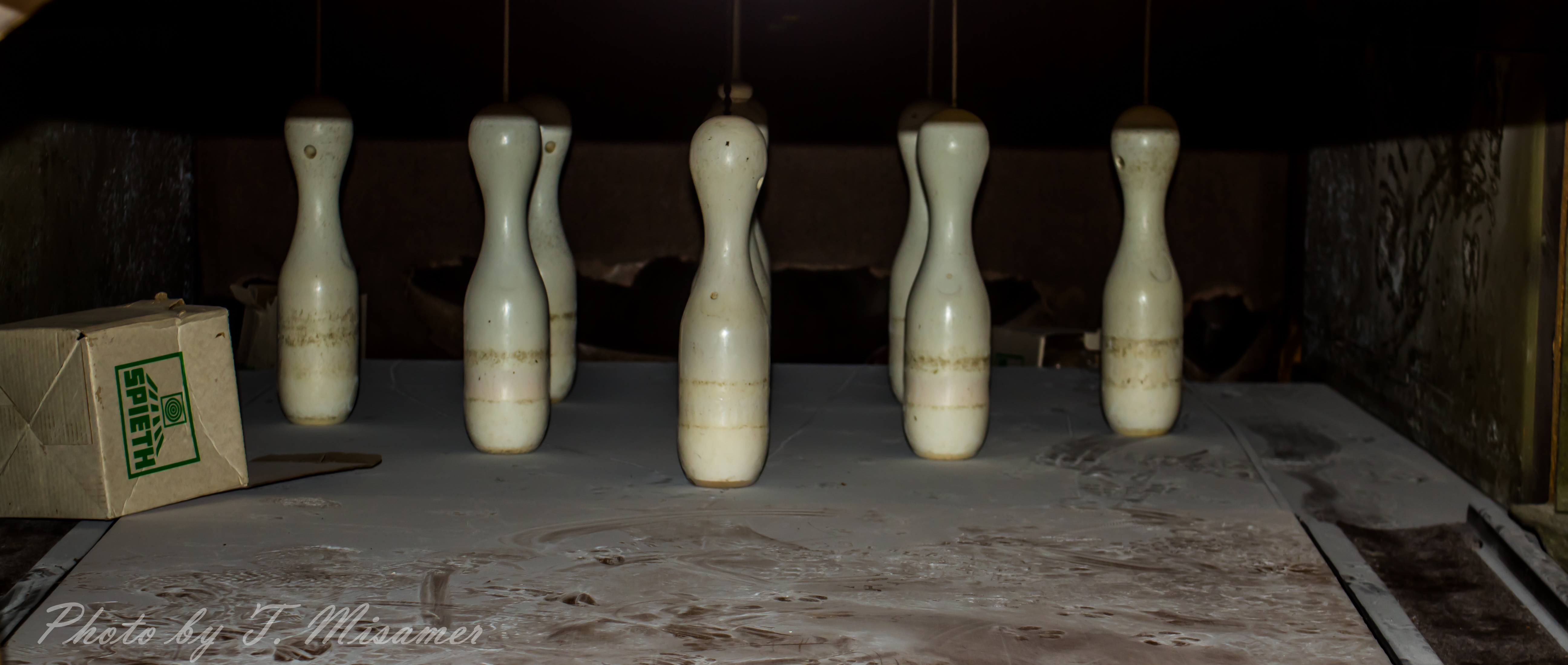This image portrays an old or possibly abandoned bowling alley, featuring a setup of unusual and seemingly cheap bowling pins. These pins appear to be made of plastic and are heavily worn, with noticeable dirt marks around their centers and discoloration at the bottoms. Each pin has a hole at the top spherical part, with pegs inserted designed to make the pins raise up when struck by a bowling ball, rather than fall over. The alley itself is incredibly dusty, indicating its long period of disuse. On the left side of the image is a dilapidated cardboard box labeled "SPIETH" in green letters, adorned with a small, indistinct symbol resembling a rounded square with a four-leaf clover design. The background is too dark to discern specific details but suggests the presence of old machinery. The entire scene conveys a sense of neglect and age, with the dusty floor and faded pins hinting at a long-forgotten past of lively games and activity.